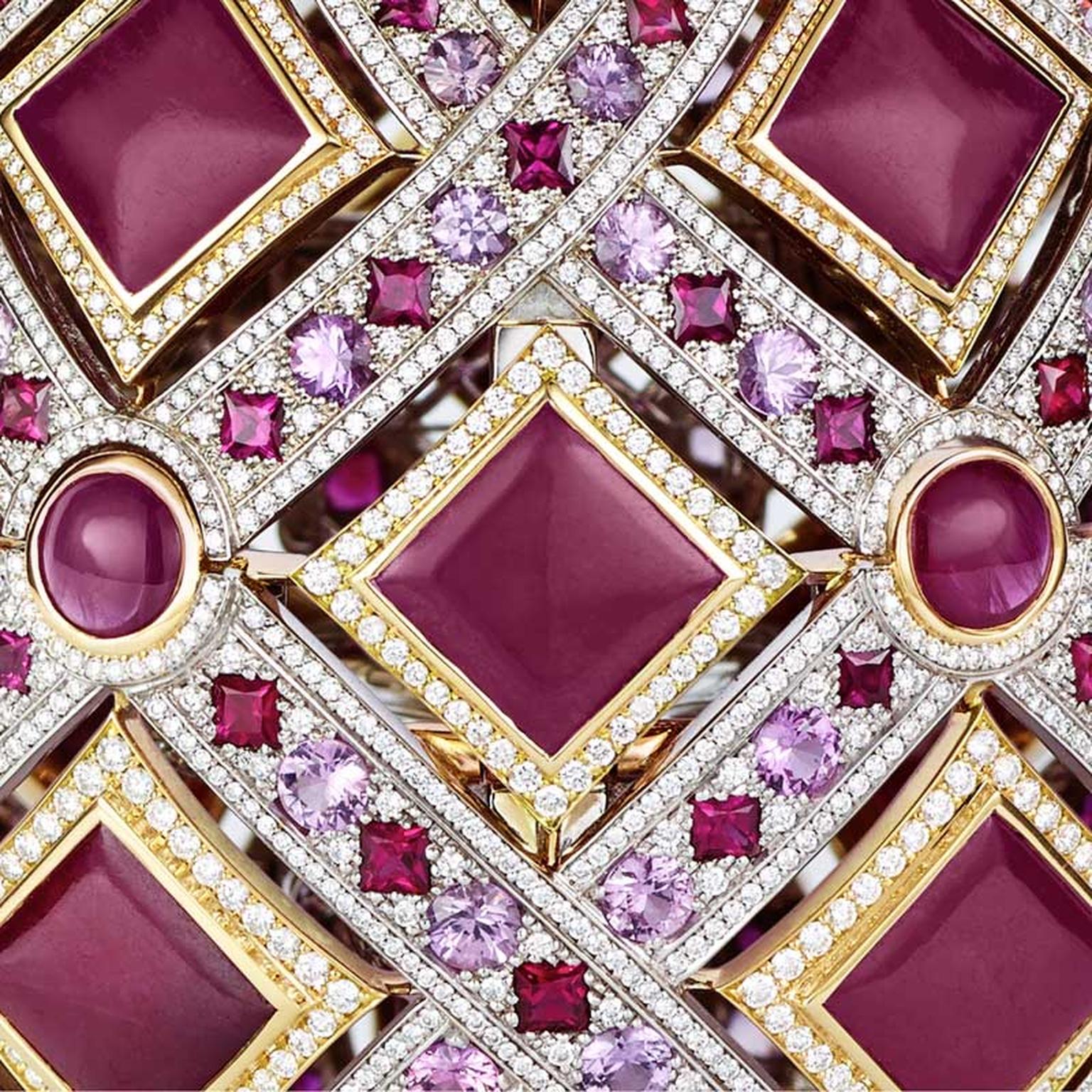The close-up photograph captures an ornate and opulent piece of jewelry, possibly part of a crown, bracelet, or headdress. The central focus features five large square gems, likely rubies or garnets, arranged in an X pattern with two at the top, two at the bottom, and one in the center. Surrounding these square gems are multiple tiny, brilliant white diamonds. Flanking the central square gem on either side are two circular gems of similar deep maroon color, each encased in gold and surrounded by more diamonds. The intricate design incorporates a lattice or crosshatch pattern with rows of alternating smaller purple and pink stones, also surrounded by diamonds. The overall craftsmanship showcases a mix of yellow gold and possibly white gold, adding a striking contrast that enhances the sparkle and color of the jewels. The combination of vibrant maroon, pale purple, and lavender stones, along with the numerous faceted diamonds, makes this piece extremely colorful and visually stunning.